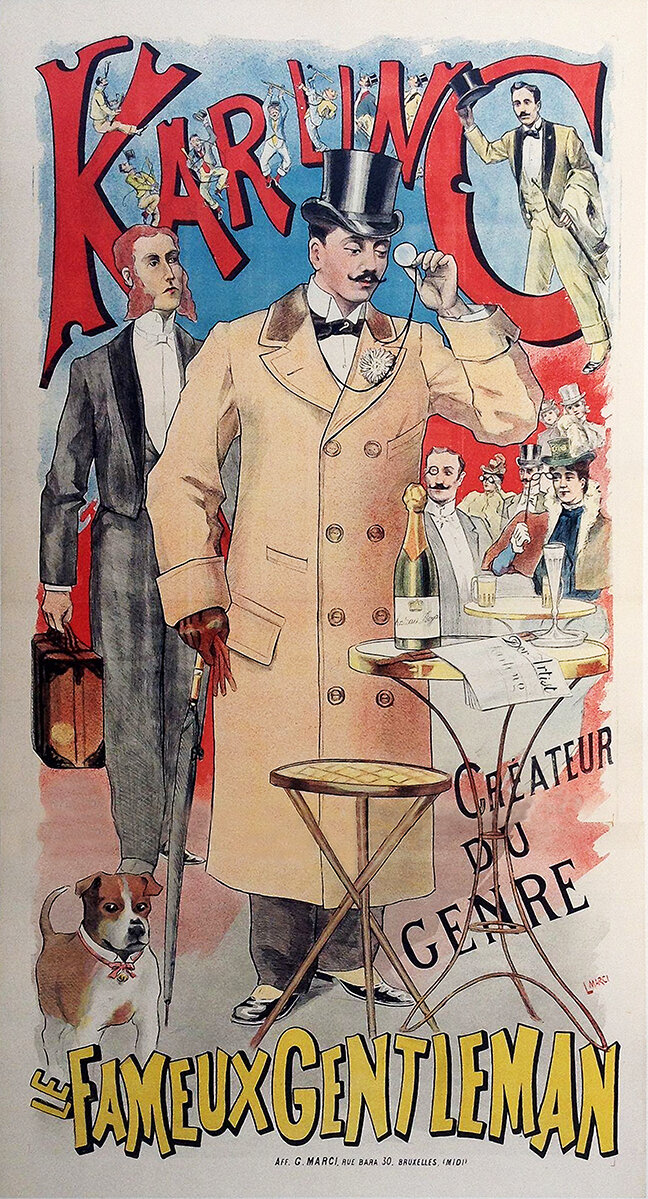This is a vintage French poster, possibly for a comic book or theatrical production, titled "Carling" in large, circus-style letters at the top. The scene is set in what appears to be an elegant setting, possibly a fancy restaurant. The central figure is a distinguished gentleman wearing a brown, double-buttoned trench coat with a fur-lined collar, a top hat, a monocle, and a bow tie. He stands by two tables adorned with a bottle of champagne, unreadable papers, and a stool. His mustache adds to his refined appearance, as he holds an umbrella and a pocket watch near his head. A small dog with a collar stands beside him.

In the background, a red-haired butler or waiter, dressed in a black suit and carrying a case, features prominently with his long sideburns. Several other similarly dressed gentlemen with old-fashioned hairstyles fill the backdrop, creating a sense of an audience or group of fellow diners. The bottom of the poster reads "Le Fameux Gentlemen," reinforcing the theme of sophistication and high society. The entire image is drawn in a cartoon watercolor style, adding a touch of whimsy to this detailed and nostalgic scene.